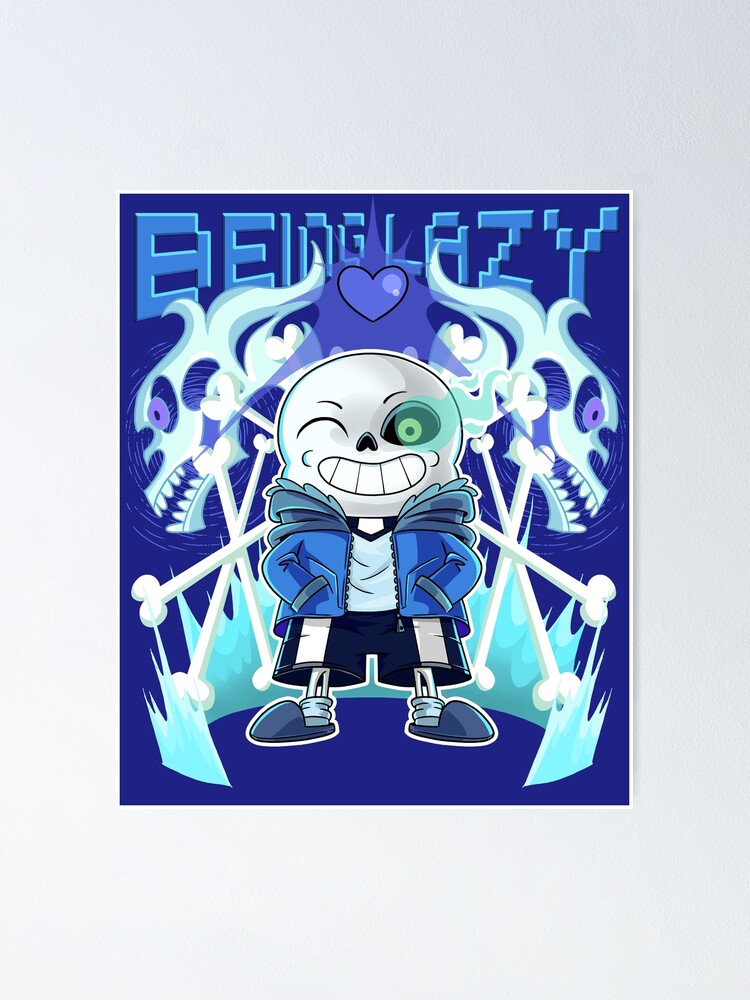The image is a computer-generated poster featuring Sans from the game Undertale, depicted in a comic book-like style. At the center of the poster is Sans, portrayed as a skeletal figure with an oversized, grinning skull. He is dressed in his iconic blue zip-up hoodie, a v-neck t-shirt, and black basketball shorts with stripes, complemented by socks and slippers. Sans' head is white, with one eye open emitting flames and a ghostly trail, and the other eye winking. His nose is heart-shaped and upside-down, with small, symmetrical eyebrows.

The background of the poster is a purplish-blue hue with a textured, pixelated effect. At the top, bold block letters spell out "Being Lazy," arranged in a way that gives a 3D perspective, drawing the viewer's eyes inward. Surrounding Sans are crisscrossed bones, creating a dynamic energy, and two spectral skulls on either side, facing outwards. Additionally, blue-tinted ice-like spikes shoot up from the ground, adding to the eerie atmosphere. Overall, the poster combines elements of horror and gaming in a visually striking manner.